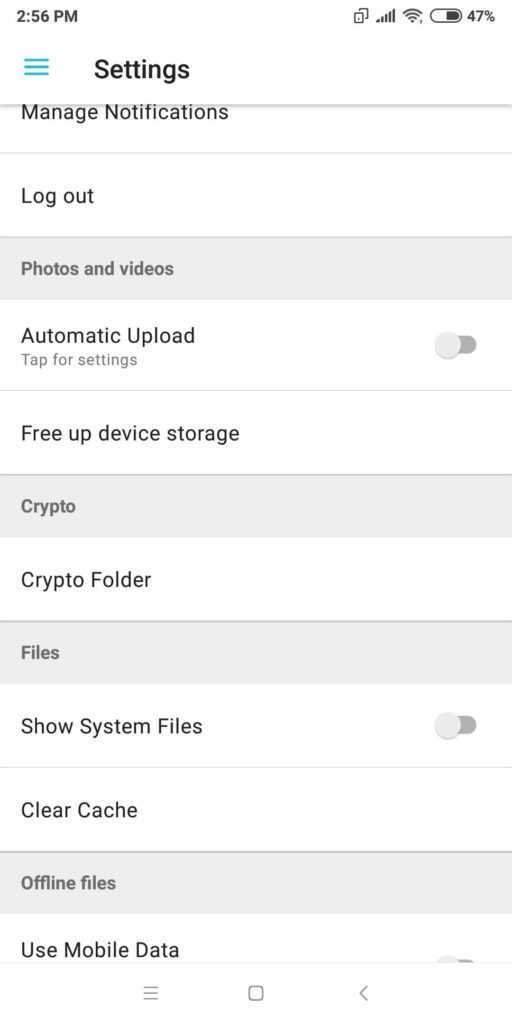The image displays a user interface on a white or light blue background. The time is 2:56 p.m., and the battery level is at 47%. At the top of the screen, there are three small blue lines and a settings icon. Below that is a major section titled "Manage Notifications," followed by an option to log out.

Next, the interface features a darker blue box labeled "Photos and Videos" and a lighter blue box with the text "Automatic Upload - Tap for Settings," accompanied by a toggle switch. Below this is an option to "Free Up Device Storage."

Further down, there's another darker blue box titled "Crypto," with a subsection labeled "Crypto Folder." Another darker blue box appears under the header "Files," which includes options like "Show System Files" with a toggle switch, and "Clear Cache."

Toward the bottom of the screen, there are options for "Offline Files" and "Use Mobile Data." The image also includes a few lines, a square, and an arrow pointing to the left, with a small dot located underneath the arrow.